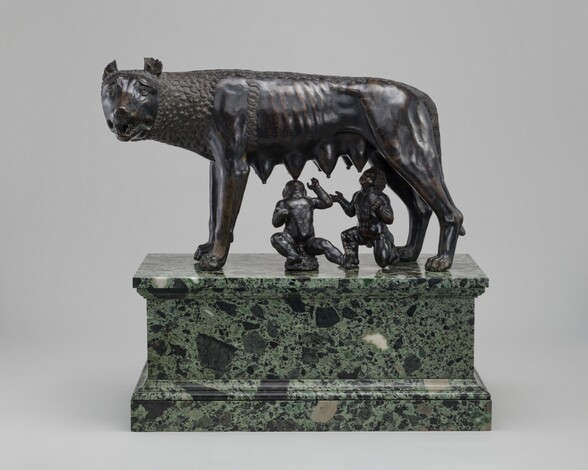The statue appears to be a black ceramic or stone figure of a wolf or a similar dog-like creature, poised on a green and black marble pedestal. The animal, with a fierce and attentive expression, gazes directly towards the observer. Disturbingly, beneath the creature, there are multiple swollen teats, seemingly full of milk. Two human-like figures, depicted in a crouched position, reach towards these teats, mouths open as if to suckle. Their hands are raised, adding to the unsettling nature of the scene. The sculpture is set against a neutral gray background, amplifying its eerie and haunting presence.